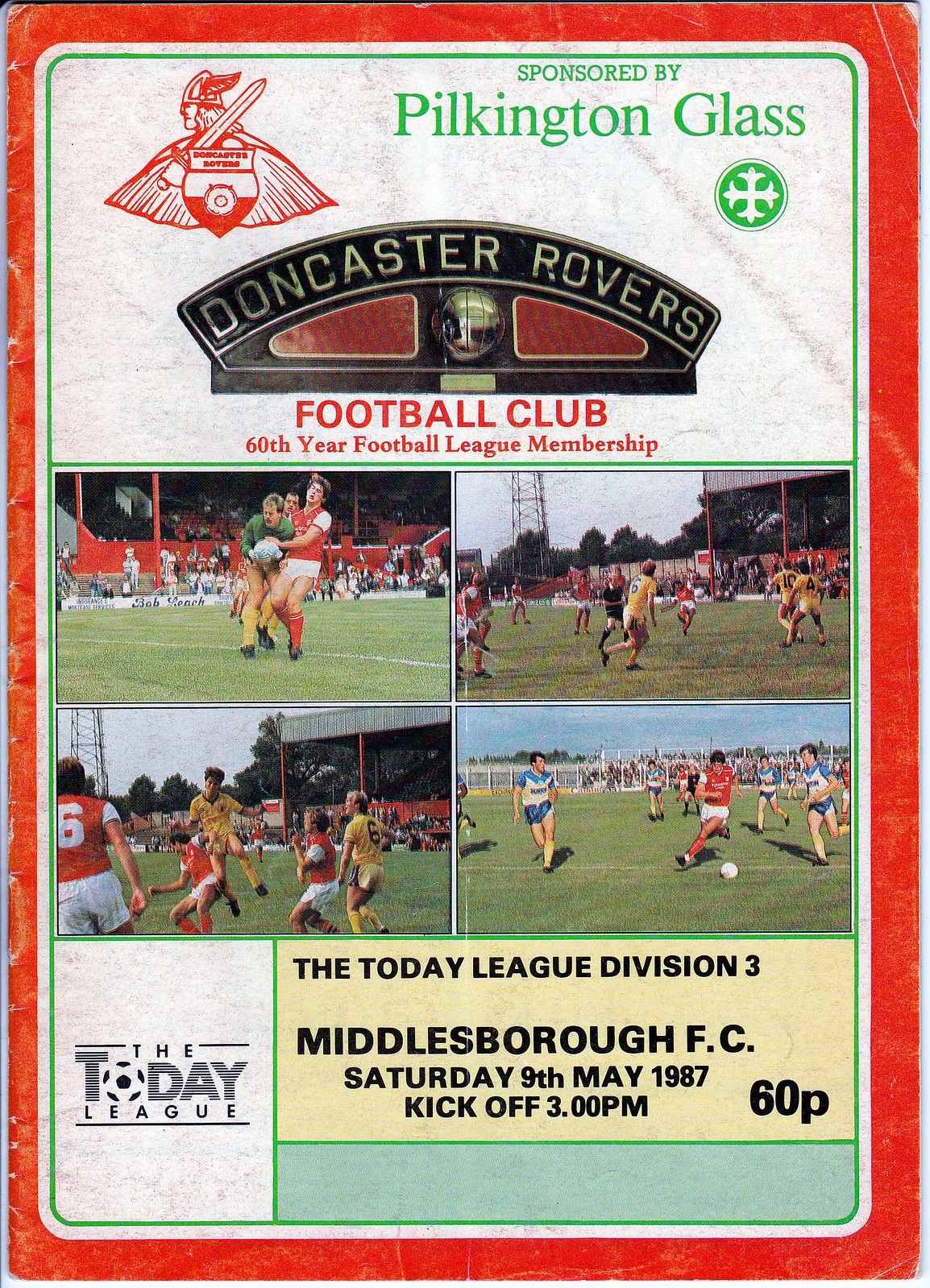This is an official program from 1987 celebrating Doncaster Rovers Football Club’s 60th year in the Football League, sponsored by Pilkington Glass. The design features a red-bordered cover with a central white background edged in green. At the top left, there's a logo depicting a Viking soldier holding a sword and shield, emblazoned with "Doncaster Rovers" in red. Centrally, the headline reads "Doncaster Rovers Football Club 60th Year Football League Membership," while below it, a collage of four pictures captures the action from a football match. The players in these images wear red jerseys with white shorts, indicating the Doncaster Rovers team, while their opponents sport yellow jerseys and shorts. The background reveals a lively crowd, electrical towers, and various stadium features like goalposts and barricades. At the bottom left corner is a logo for "The Today League" with the 'O' stylized as a football, and on the right side, a text box details, "The Today League, Division III, Middlesboro FC, Saturday, 9th of May, 1987, Kickoff 3 p.m., 60p."